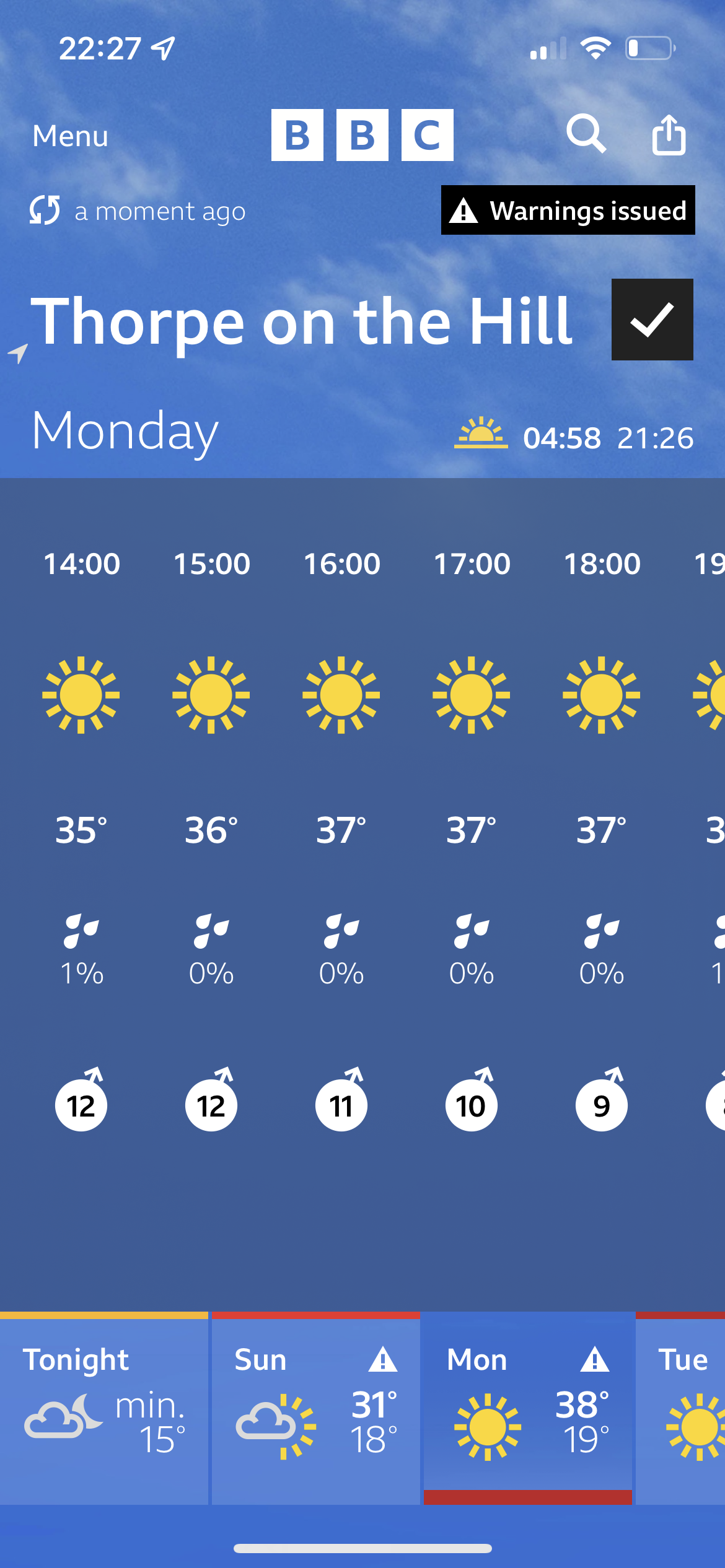This image is a detailed screenshot from a BBC weather app on someone's phone displaying the weather forecast for Thorpe on the Hill. At the top of the image, the time reads 22:27, with Wi-Fi and a battery icon at 25%. The header features a blue sky with dustings of clouds. It displays various icons and text including "Menu," "BBC," a search magnifying glass, and a refresh button labeled "a moment ago." Prominent black-highlighted warnings display "warnings issued" with a triangle and exclamation mark, and the location "Thorpe on the Hill" is listed above a black square with a white checkmark. Below this, "Monday," "04:58," and "2126" are shown beside a sun icon.

The main section of the image has a dark blue background, broken into columns showing hourly forecasts from 1400 to 1900 hours. Each hour is marked by a sun icon, temperatures ranging from 35°C to 37°C, a 0-1% chance of rain, and wind gusts denoted by white circles with arrows (values ranging from 9 to 12). 

The footer elaborates on the weather for the coming days with blue-colored sections for each day: 
- "Tonight" features a moon and cloud icon, indicating a minimum of 15°C.
- "Sunday" shows a cloud with sun rays, forecasting 31°C during the day and 18°C at night.
- "Monday" displays a fully sunny icon with highs of 38°C and lows of 19°C.
- "Tuesday" is partially visible, showing another fully sunny icon. 

This detailed display combines temperatures, visual conditions, and additional weather information to provide a comprehensive local weather forecast.